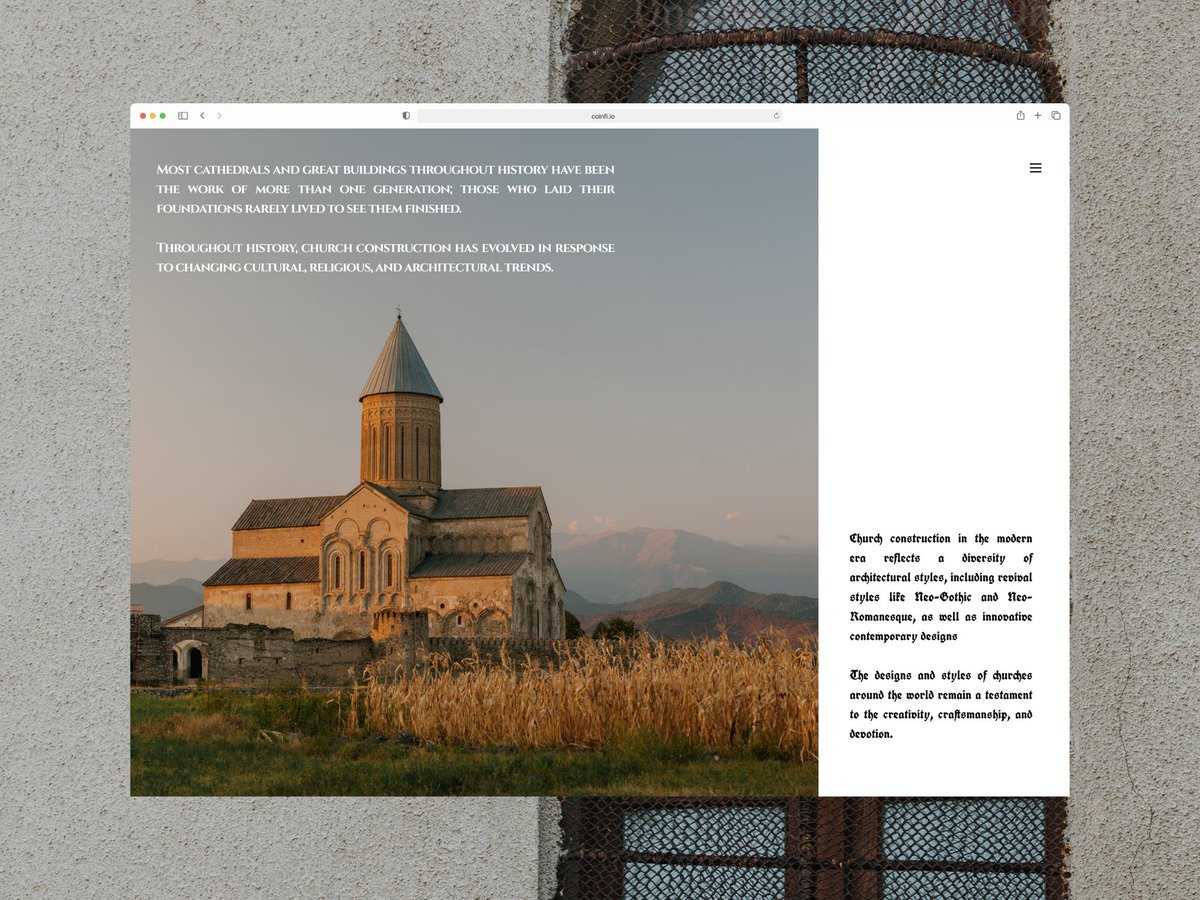This image displays a Mac-style computer desktop with a distinct background featuring a rusted chain link mesh against a cement backdrop, reminiscent of an urban environment. Central to the image is a window that resembles a webpage or a flyer, with visible Mac Explorer controls at the top, indicative of an Apple operating system.

The main content of this window showcases a scenic depiction of a grassy field, dotted with what appear to be tall corn stalks on the right. In the background, rolling hills lead up to a prominent stone church, rendered in a classic medieval architectural style, standing majestically under a gray sky. Superimposed on this scene is white text that reads: "Most cathedrals and great buildings throughout history have been the work of more than one generation. Those who laid their foundations rarely lived to see them finished. Throughout history, church construction has evolved in response to changing cultural, religious, and architectural trends."

To the right side of the window, there is a white strip containing additional text stating: "Church construction in the modern era reflects a diversity of architectural styles including revival styles like neo-Gothic and neo-Romanesque as well as innovative contemporary designs. The designs and styles of churches around the world remain a testament to the creativity, craftsmanship, and devotion."

This detailed image captures the juxtaposition of modern technology with historical architectural reflections, emphasizing the evolutionary journey of church architecture through various cultural and stylistic influences.